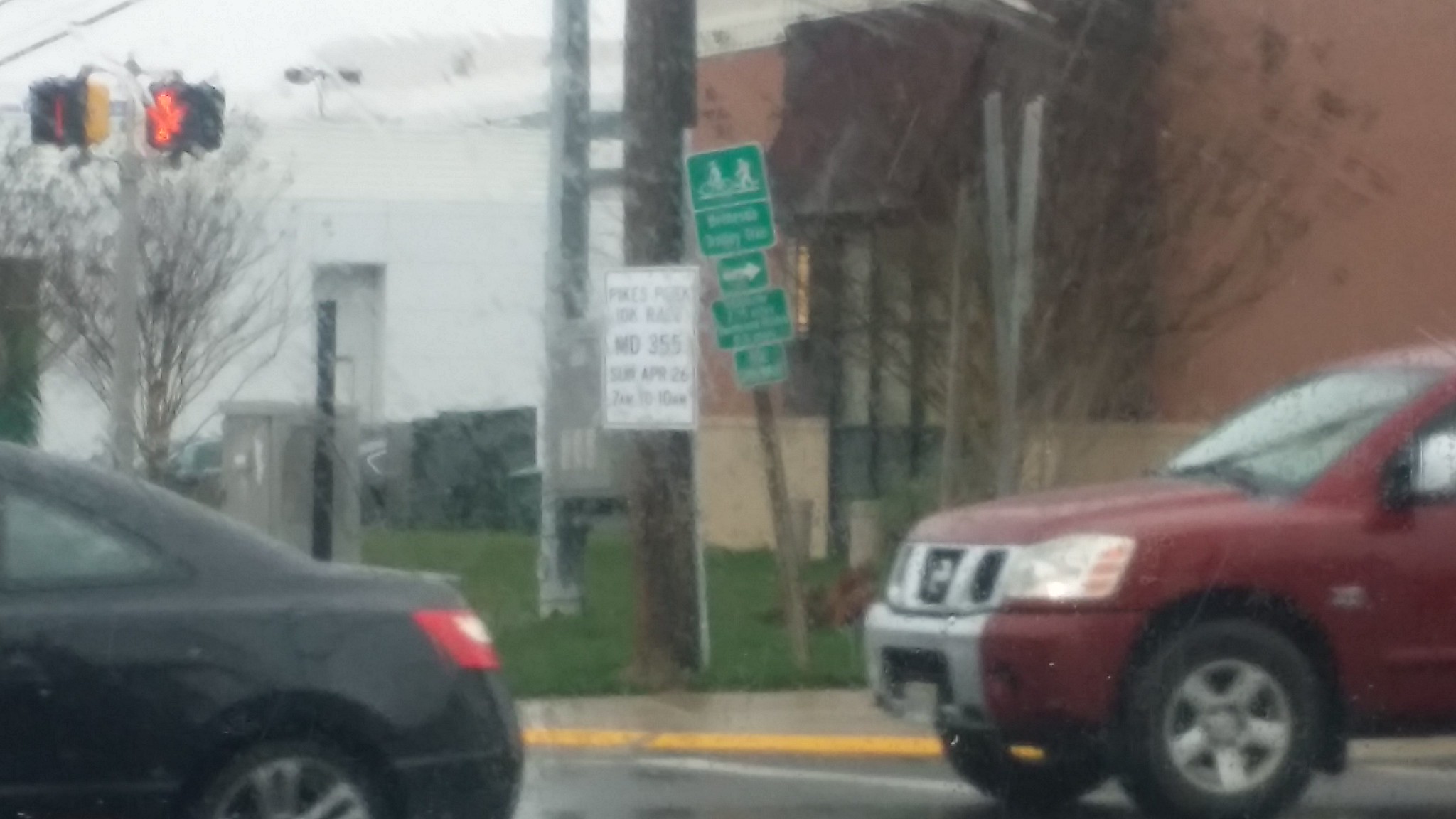This blurry photograph captures a dreary street scene with overcast skies, suggesting a rainy or windy day. In the foreground, the rear end of a black sedan with its red tail lights is visible, occupying the lower left portion of the image. Behind it, the front end of a red SUV or larger vehicle with a silver grille is seen. The vehicles are parked on a black asphalt street edged by a yellow curb.

In the middle ground, a series of signs appear: a white sign and a green sign mounted on a pole, along with another pole featuring multiple green signs with white writing. A leaning directional sign can also be spotted. On the right side of the scene, there's a short, brownish brick building with windows and a brown awning extending over the sidewalk. 

In the background, near the top left of the image, streetlights and traffic lights with yellow backgrounds and red signals are visible against the light gray, cloudy sky. A tree with no leaves stands near the brick building, adding to the somber atmosphere of the photograph.